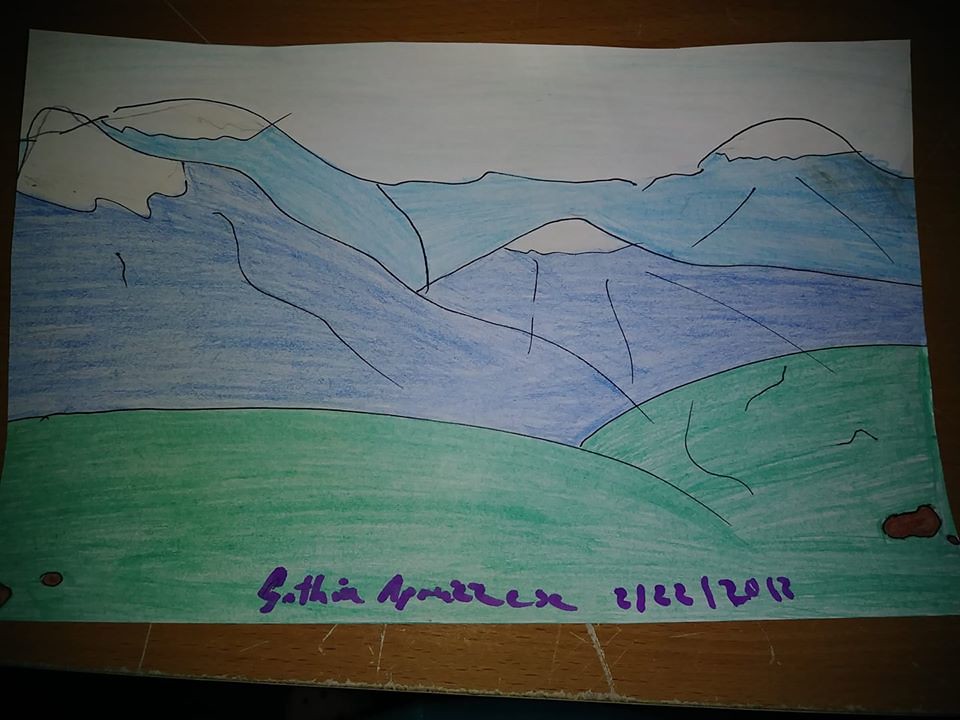This photograph shows a drawing on a piece of white printer paper, placed on a scratched, wooden tabletop. The drawing depicts a mountainous landscape, intricately detailed with various media, including pen and colored pencils. The foreground features a lush green grassy area, with some brown rounded objects scattered across it. Behind this are two dark-colored mountains with prominent white snowcaps, drawn primarily in black pen. Further back, there is a range of blue and purple mountains, also capped with white. The sky is subtly rendered with very light streaks of blue and white, giving it a delicate appearance. At the very bottom of the drawing, there is an artist's signature, difficult to decipher, which appears to be written in purple marker. The legible date next to the signature is either 2-22-2012 or 2-22-2013. The overall presentation is a slightly dim, well-worn, yet charming snapshot of creativity.